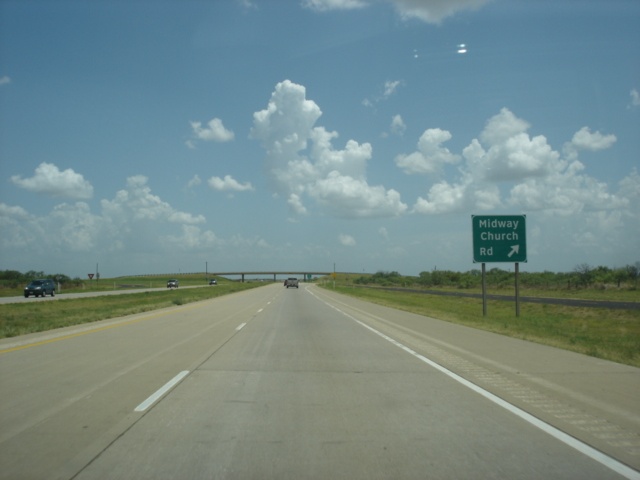The outdoor photograph captures a two-lane highway taken from the viewpoint of a vehicle traveling along it. The asphalt highway, characterized by a center dotted white line and a solid line on the right, descends into the distance towards a horizon marked by a bridge or overpass. The highway is flanked on its left by a grassy median strip, separating it from the opposing traffic lanes filled with oncoming cars. On the far right, there's a grassy area featuring a roadside sign, mounted on two metal poles, which reads "Midway Church Road" in white letters on a green background, with an upward right-pointing arrow at the lower right corner of the sign.

Further up the highway, several cars are visible heading towards the bridge that spans the horizon. Beyond the bridge, the horizon line is punctuated by tree lines. Dominating the upper half of the image is a vibrant, dark blue sky that gradates to a light gray closer to the horizon, adorned with puffy white clouds. A service road, darker than the main highway, can also be seen on the extreme right, accompanied by additional tree lines.